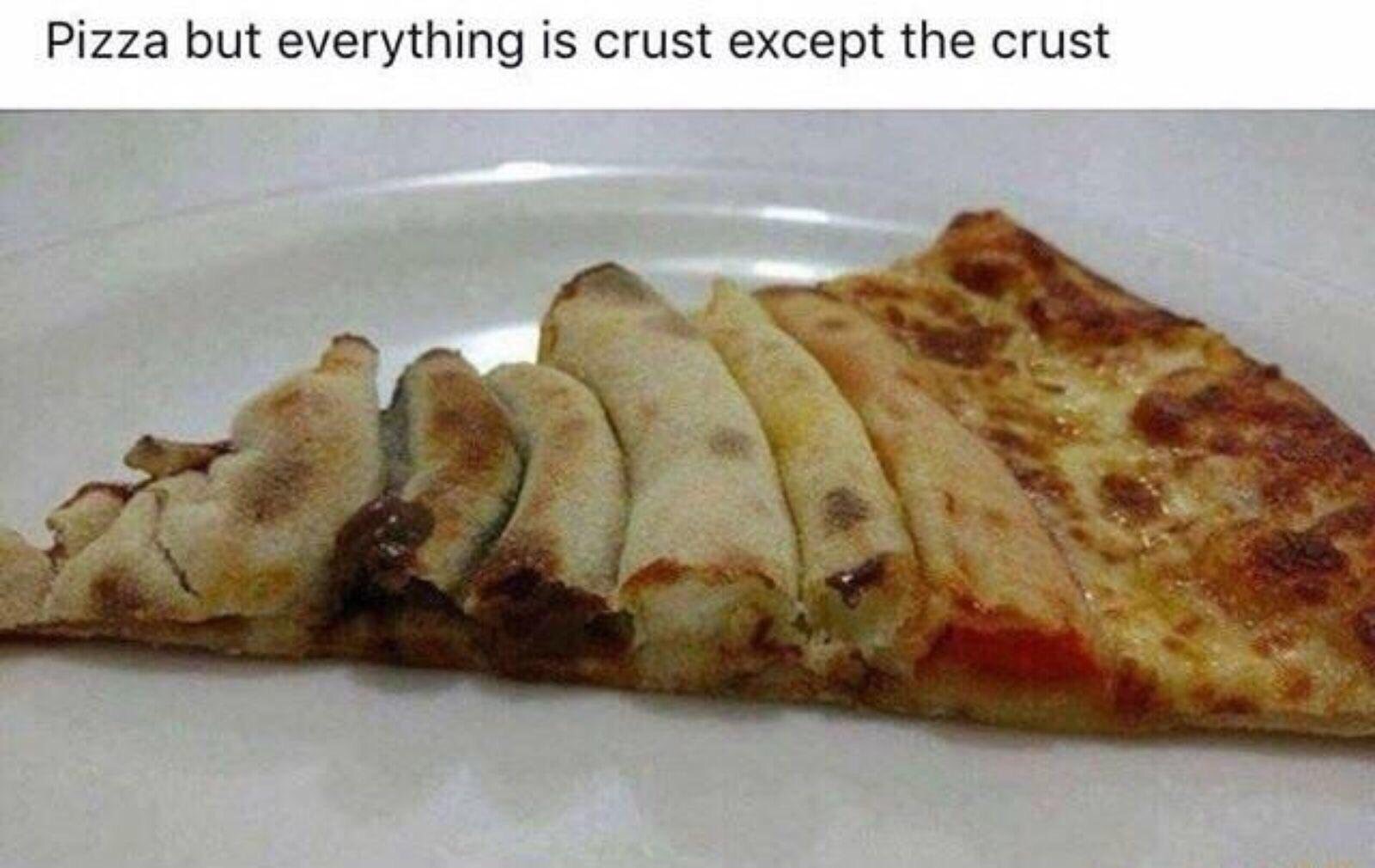The image showcases a creatively reimagined slice of pizza placed on a white plate against a white backdrop. The photo is captioned above in black text: "Pizza, but everything is crust except the crust." This unique pizza slice has been cleverly assembled to reverse the typical pizza structure. The usual crust perimeter is replaced with melted cheese and a hint of sauce, while the main body of the slice is formed by several tube-like structures of pizza crust, meticulously arranged either horizontally or vertically. This inventive setup results in approximately three-fourths of the slice being composed of crust, with no traditional toppings like pepperoni in sight. The crusts are browned to perfection, adding an interesting twist to an iconic dish.